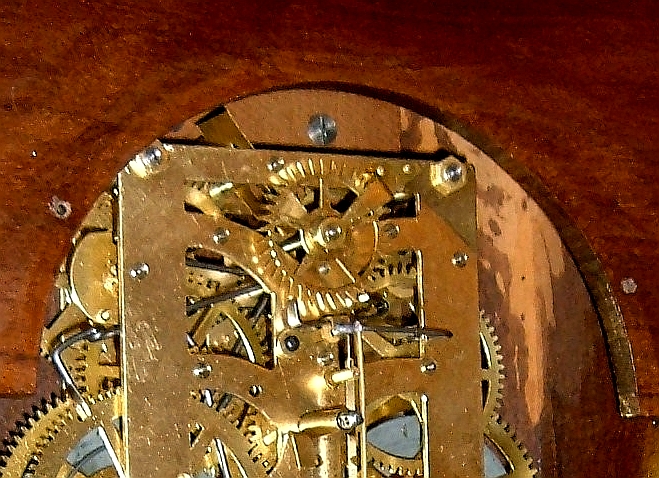The image depicts the intricate inner workings of a clock, primarily featuring components in gold, brass, and silver. The large, interconnected gear wheels and smaller rotary elements dominate the scene, set against a backdrop of reddish wooden panels. The clockwork itself is primarily golden, with numerous silver screws and bolts securing the various parts. Notably, some darker, gray screws also contribute to the intricate assembly. The wooden structure, which arches at the top, shows signs of wear with light dings, nicks, and possible water damage that has slightly stripped away the finish. The flash of the camera accentuates the metallic sheen of the clockwork. Overall, the detailed mechanical components, combined with the ornate yet weathered wooden enclosure, convey the complexity and age of this remarkable timepiece, viewed from its backside rather than its face.